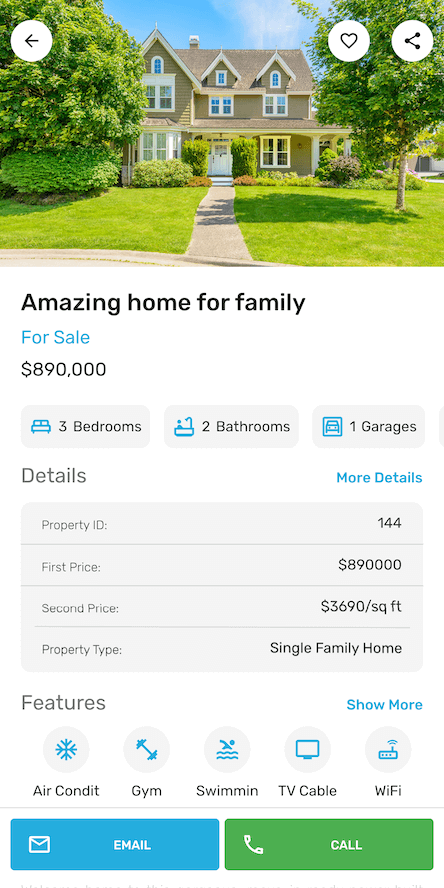The image appears to be taken from a cell phone interface, though it lacks the usual status indicators such as the battery level, signal bars, and time. Instead, it features three circular icons at the top of the screen against a white background with black writing. The leftmost circle contains a backward arrow key, the rightmost circle has a heart icon, and to the far right, there's a share button.

The displayed image occupies the top quarter of the screen and depicts a tan-colored house with a manicured front yard featuring trees and a sidewalk leading up to the front door. The trees cast shadows on the yard, suggesting a sunny day.

Below the image, bold black text reads "Amazing home for family." Underneath, in blue text, it states "For Sale." The price of the house is listed in black writing as "890,000." Further details about the house are provided in three bullet points: 
- Three bedrooms
- Two bathrooms
- One garage

Below these specifics, the section titled "Details" lists additional information such as property ID, first price, second price, and property type. 

At the bottom of the screen, various features of the house are itemized: air conditioning, gym, swimming pool, TV cable, and Wi-Fi. 

Finally, there are two interactive buttons: a blue box on the left with white writing and an email icon labeled "Email," and a green box on the right with white writing and a telephone icon labeled "Call."